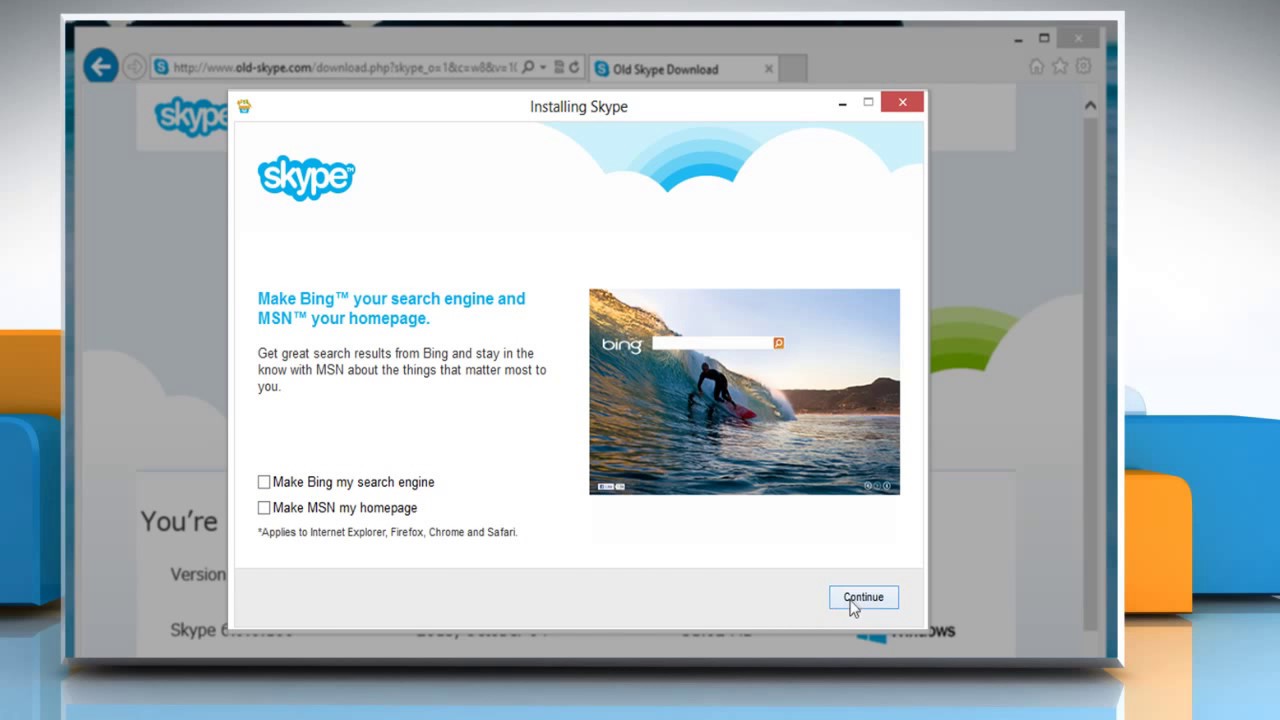The photograph, likely sourced from the Skype website, serves instructional purposes. Framed by left and right borders, the image centers on a computer monitor screen, though only the screen is visible. Displayed on this screen is a page from the Skype website, slightly grayed out to highlight a white pop-up box in the center. This pop-up box is part of the Skype installation process, as indicated by the text "Installing Skype" at the top. Positioned in the upper left corner of the pop-up is the Skype logo, presented in lowercase white letters outlined in sky blue.

Below the logo, the message "Make Bing your search engine and MSN your homepage" is written in sky blue font. Adjacent to this text, on the right, is a visual from the Bing homepage, showcasing a stunning photograph of ocean waves with a surfer near the shore, mountains in the background, and a beautiful sky above. At the lower left of the pop-up, a checkbox option allows users to select "Make Bing my search engine, make MSN my homepage." In the lower right corner, a gray button labeled "Continue" invites the user to proceed.